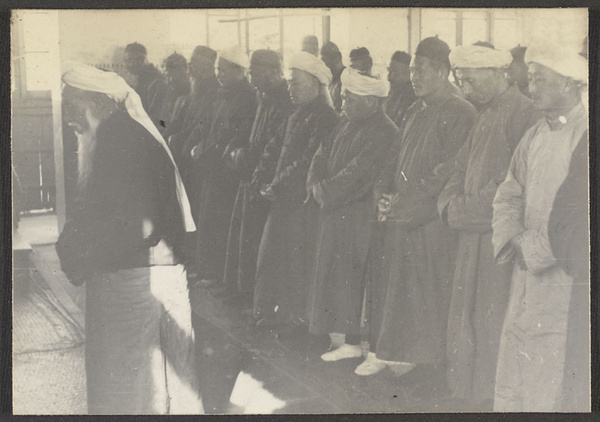This aged, sepia-toned photograph, now yellowed with time, depicts a group of men standing on a wooden floor, possibly within a religious setting such as a mosque, which is suggested by their barefootedness. The men, who seem to belong to an Asian ethnicity—potentially Chinese, Indian, or Tibetan—are all wearing traditional, long coats in varying shades of gray. Their hands are clasped at their waists, indicating a prayerful stance. Each man has a form of head covering, ranging from white turbans to fez-like caps. A notable figure stands at the forefront on the left: an elder with a thick white beard, wrapped in a head cloth that drapes over his back, clad in a black shirt and skirt-like garment. This man appears to be a spiritual leader, with numerous others—possibly students or disciples—standing behind him, following a similar dress code. The image conveys a strong sense of cultural and spiritual unity amidst an atmosphere of contemplation and solemn devotion.